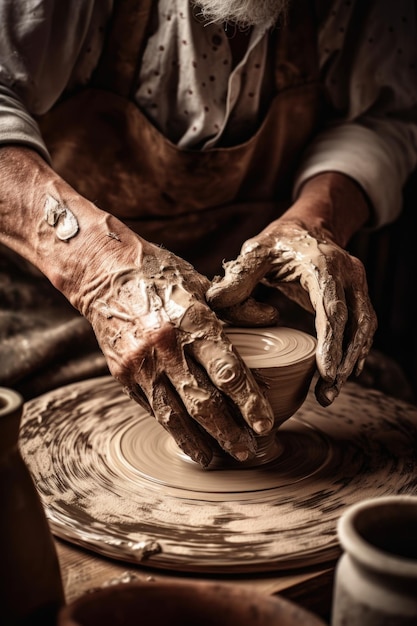A close-up photograph captures the meticulous hands of an elderly artisan skillfully molding wet clay on a spinning potter's wheel. The hands, with their aged texture and experience, are centered as they shape a small mass of clay that glistens with moisture, reflecting the ambient light. The motion of the wheel is evident in the concentric, blurred lines around the clay, indicating a dynamic creation process. The worker's sleeves are rolled up to the forearms, revealing a grey shirt beneath a brown apron, suggesting a pragmatically dressed potter at work. The top portion of the image hints at a bearded man, though his face remains obscured, focusing the viewer's attention on the masterful manipulation of the clay. The background and foreground contain elements of the potter's environment, with out-of-focus clay pots and tools that contextualize the scene without detracting from the central activity of the wheel and the craftsman's hands.